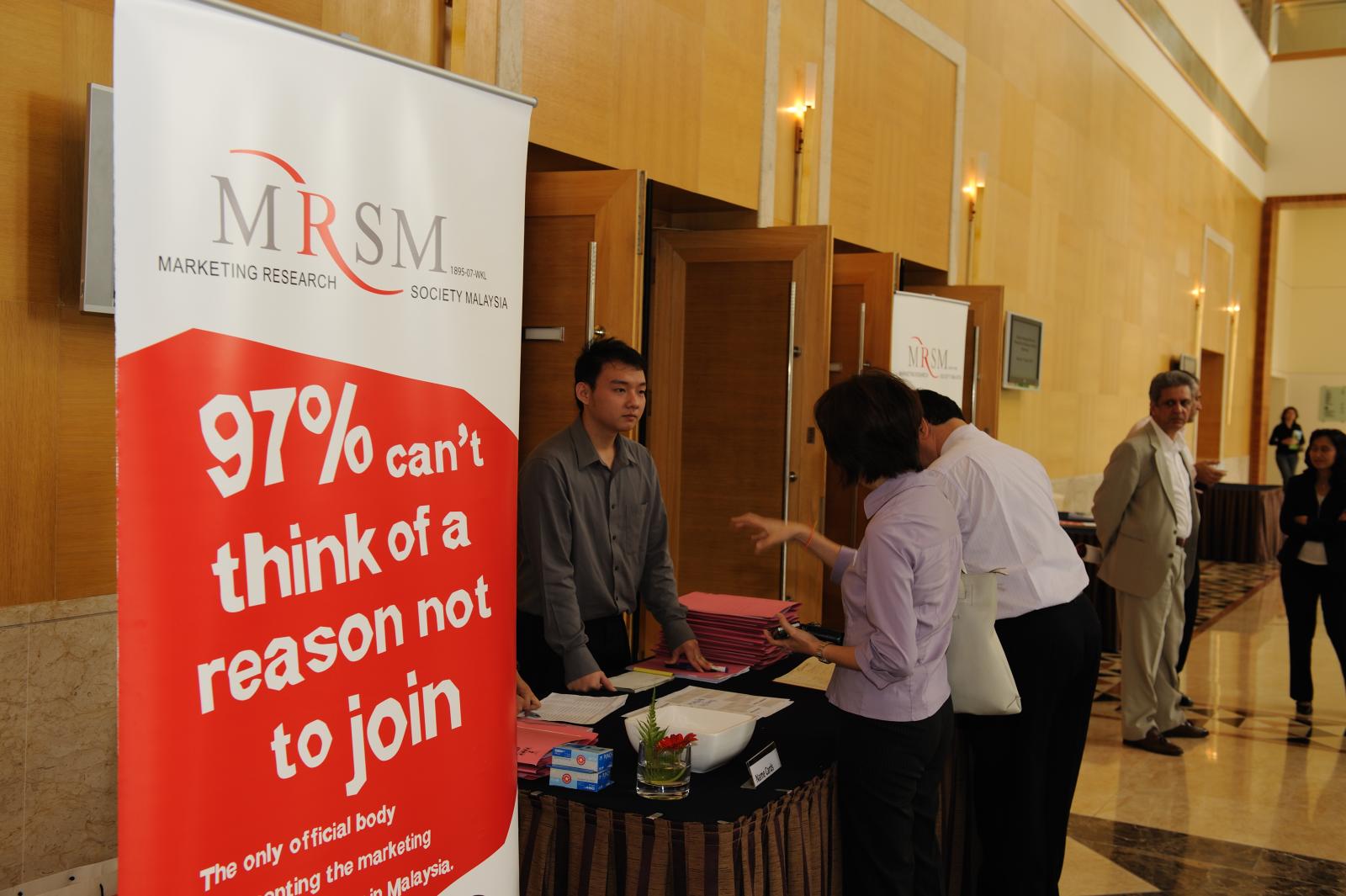In the photograph of an indoor setting, we see a young Asian man in a long-sleeved button-up gray shirt standing behind a table with a black top and brown skirt. The table, located roughly in the center of the image, is adorned with various papers, books, a vase with a flower, and a stack of pink folders. On the left side of the image, a large rectangular banner stands out, displaying the text: "MRSM, Marketing Research Society of Malaysia" with the phrase "97% can't think of a reason not to join" in white letters over a red background. The floors are a mix of light gray and brown tiles, and the walls are done in light wood paneling, featuring small light sconces that emit a warm orangish or yellowish glow.

Two individuals on the right side of the table engage with the young man, looking over the documents. In the background, four other people are visible, dressed in business formal attire, suggesting a professional setting, possibly a conference or convention. Various tables line the wall, adding to the impression of an organized event space. The darker-colored doors behind the central figure frame the scene, enhancing the structured aesthetic of the setting.